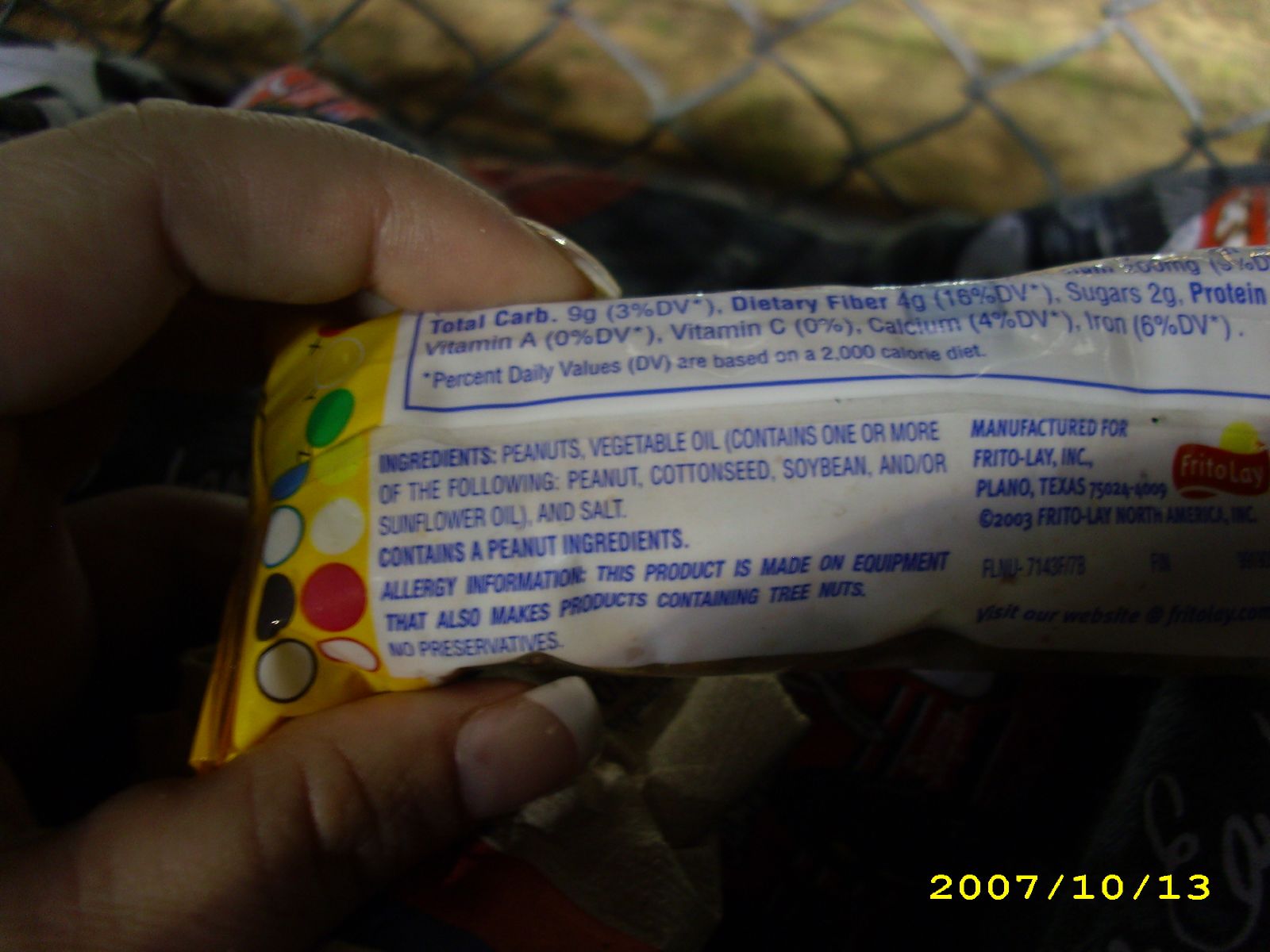This photograph is a detailed close-up of the back of a rectangular, yellow and white candy wrapper, held by a woman's left hand. The left side of the wrapper features a yellow section adorned with multicolored circles—green, red, white, blue, yellow, and black. The center showcases the nutritional information and ingredients in blue text set against a white background. The text "manufactured for Frito-Lay, INC, Plano, Texas" is visible towards the right side. At the bottom right of the image is a date mark, "2007-10-13," in yellow. The scene is set against the backdrop of a gray chain-link fence with some grass visible through it. Additionally, the hand holding the wrapper rests on gray fabric flecked with white and red.